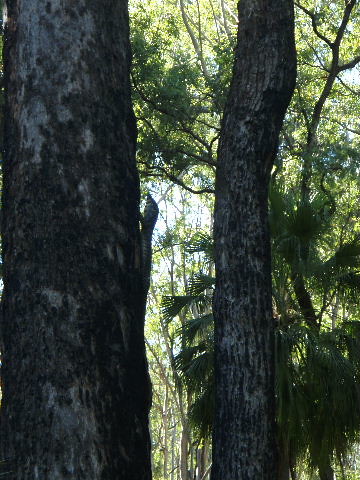In this outdoor scene of a forest, the image captures a dense, wooded area bathed in daylight. Dominating the left side of the picture is a large, weathered tree trunk, marked by dark gray and lighter gray patches where the bark is chipped and worn from the elements. This trunk extends out of the frame, its top obscured from view. To its right and slightly behind, another tall tree trunk stands with a similar but less weathered appearance, exhibiting a gray and black color mix. Further right, in the mid-ground, a smaller tree with fern-like green leaves juts up, its thin trunk splitting into various branches. The background is filled with a multitude of trees, some bare and some adorned with leaves. The sun illuminates the distant foliage, contrasting with the shadowed foreground, where the large trunks reside. High above, glimpses of a blue sky peek through, suggesting broad daylight despite the shadowy depth of the forest. Additionally, there appears to be a silhouette of something, possibly a lizard or another branch, crawling up the large trunk on the left.